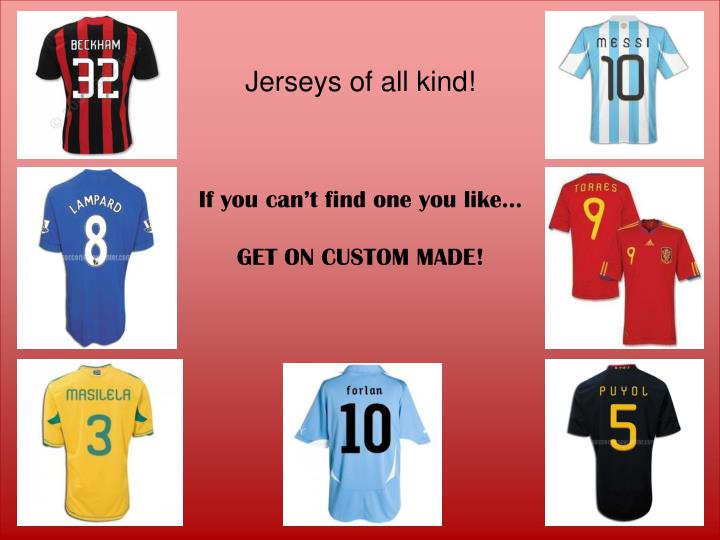The advertisement showcases a variety of jerseys against a striking background that transitions from dark rose at the bottom to a lighter shade at the top. At the center of this background, a bold black font declares “Jerseys of all kinds!" Below this, in a smaller font, the tagline reads, “If you can’t find one you like… get one custom made!”

On the left side of the ad, three jerseys are displayed vertically: a red and black jersey with "Beckham 32," a blue jersey with "Lampard 8," and a yellow jersey with "Masekela Lila 3" in green font. Centrally, at the bottom of the ad, there is a navy jersey with "Follin 10." The right side features three more jerseys arranged vertically: a blue-striped jersey with "Messi 10," a red jersey with "Torres 9" in yellow font, and a black jersey with "Puyol 5."

The overall layout is visually engaging, with the gradient background enhancing the colorful assortment of jerseys. Thin, dark red borders encircle the ad, giving it a polished finish. The consistent emphasis on names and numbers along with the diverse color palette effectively highlights the variety and customization options available.